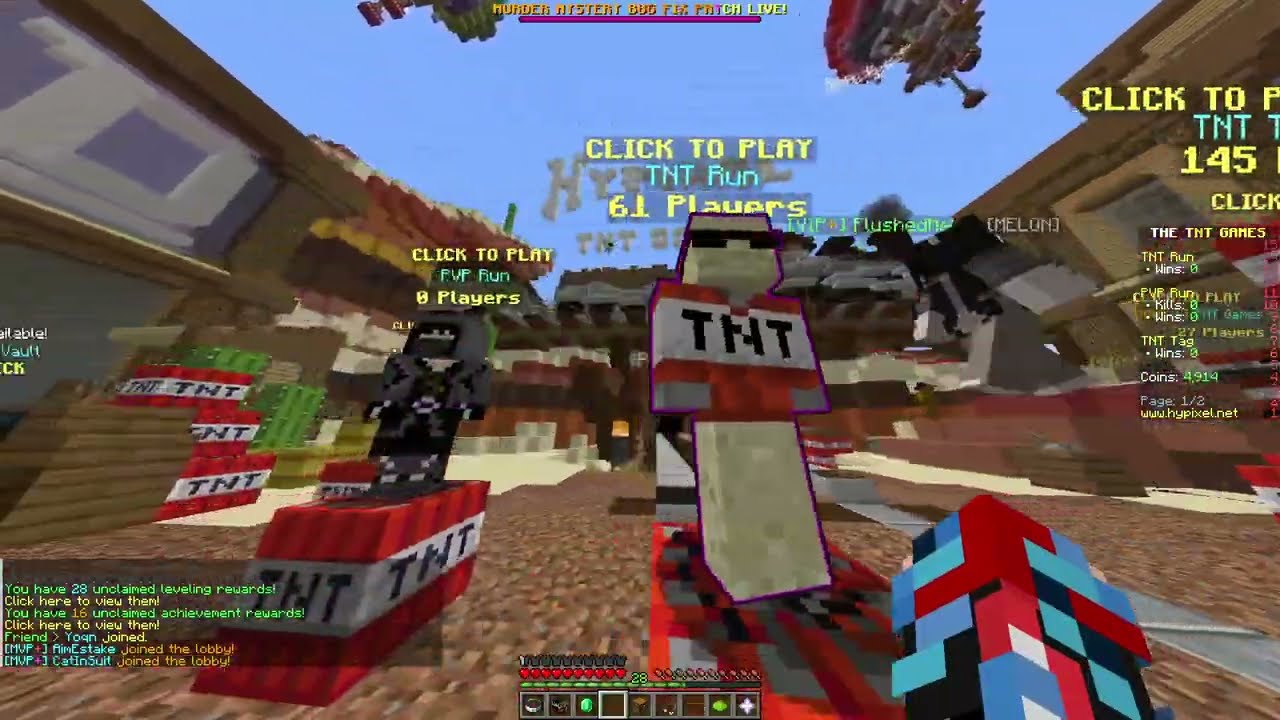In this detailed screenshot from a video game that borrows heavily from Minecraft's iconic blocky aesthetics, the scene reveals a bustling multiplayer arena named "TNT Run" with 61 active players. Dominating the foreground is a character in a red shirt emblazoned with a white stripe and black "TNT" text. This character sports black sunglasses and stands atop a pile of red dynamite blocks marked similarly with "TNT." To the left, another character dressed in a black cloak and mask, resembling a ninja, also stands on a pile of TNT. Both figures are set against a backdrop of brownish stone walls and scattered cobblestone paths that outline a small, chaotic village environment. Various on-screen texts add to the clutter: prominently, "Click to play TNT Run, 61 players" sprawls across the middle, while additional options, such as "Click to play PvP Run, 0 players," and numerous chat messages about unclaimed rewards and lobby joins, litter the bottom and left of the screen. The pale blue sky at the top enhances the game's familiar pixelated charm.